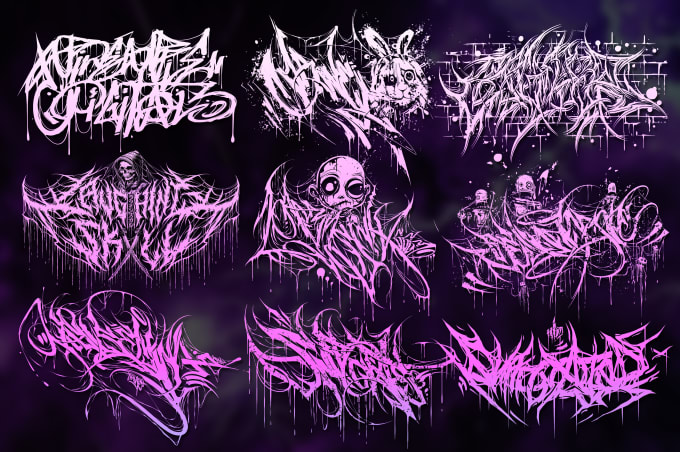This color illustration showcases a vibrant graffiti art piece set against a predominantly dark background with some gradient soft purple and green tones. The artwork is organized into a grid with three rows and three columns, totaling nine distinct pieces. The graffiti in the top row features light colors, predominantly soft pinks and almost white hues with some drip marks, with the central piece displaying a rabbit shape to the right side. The middle row incorporates slightly darker pinks; the first piece on the left prominently shows a Grim Reaper figure, while the central piece features an alien head. The bottom row is characterized by bright, vibrant pinks and purples. The combined elements of New Funk and New Metal styles lend a unique and edgy vibe to the overall image, making each piece stand out with intricate yet somewhat illegible text forms.